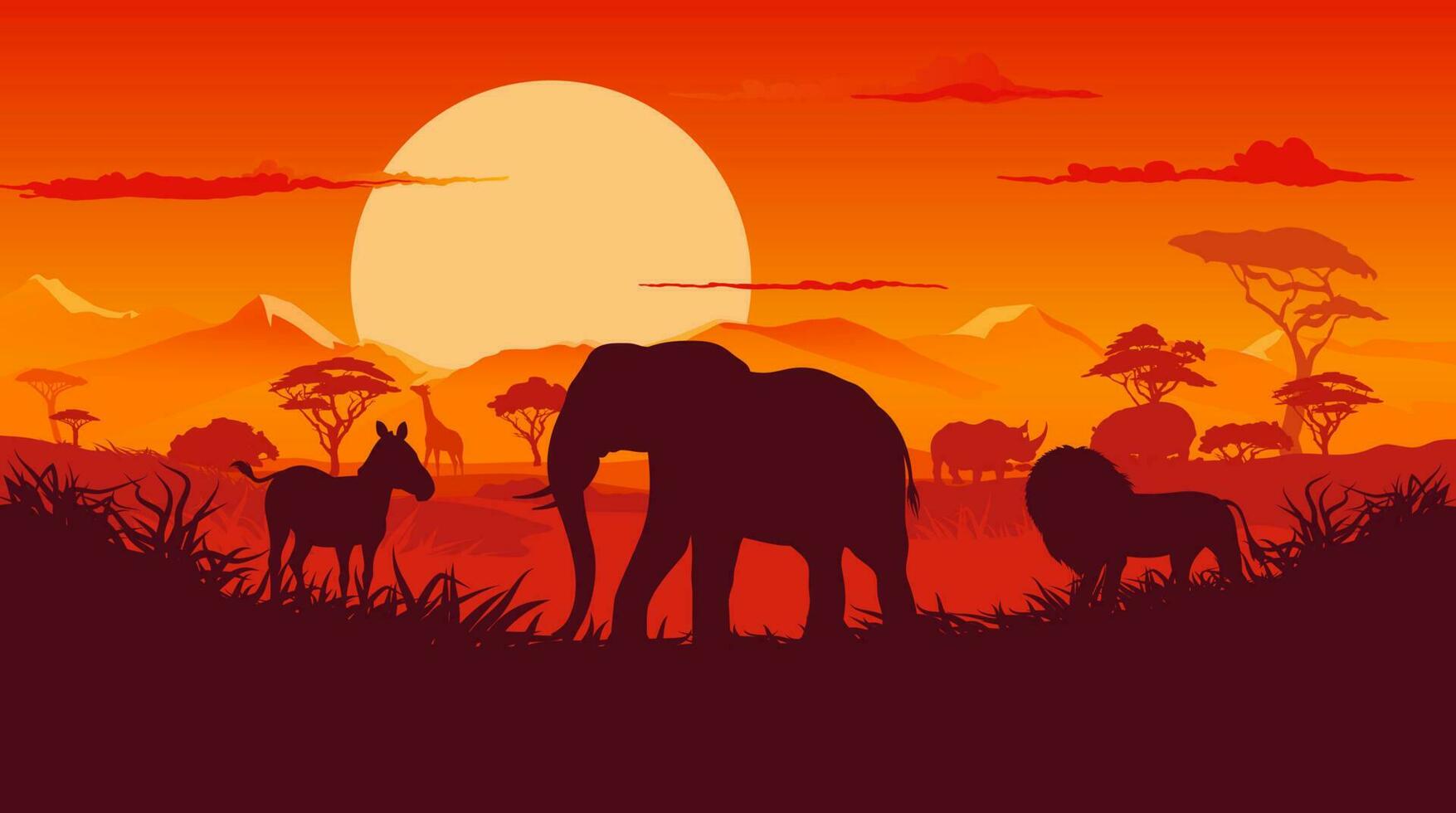The illustration captures a vibrant and stunning scene of the African savanna at sunset, reminiscent of a scene from "The Lion King." In the foreground, black silhouettes of grass form a semicircle, framing the central figures: an elephant facing left, a lion facing left, and a zebra facing right. The background is layered with silhouettes in varying shades of brownish-red, depicting a giraffe, rhinoceros, and hippopotamus, along with several trees. Further back, majestic mountain ranges appear in shades of light and dark orange. Dominating the sky is a large, pale yellow sun, framed by the rich red-to-orange gradient of a beautiful African sunset, with thin, dark orange clouds hovering above the mountains. The overall composition, though cartoonish, deeply resonates with the exotic beauty and warmth of the African wilderness.